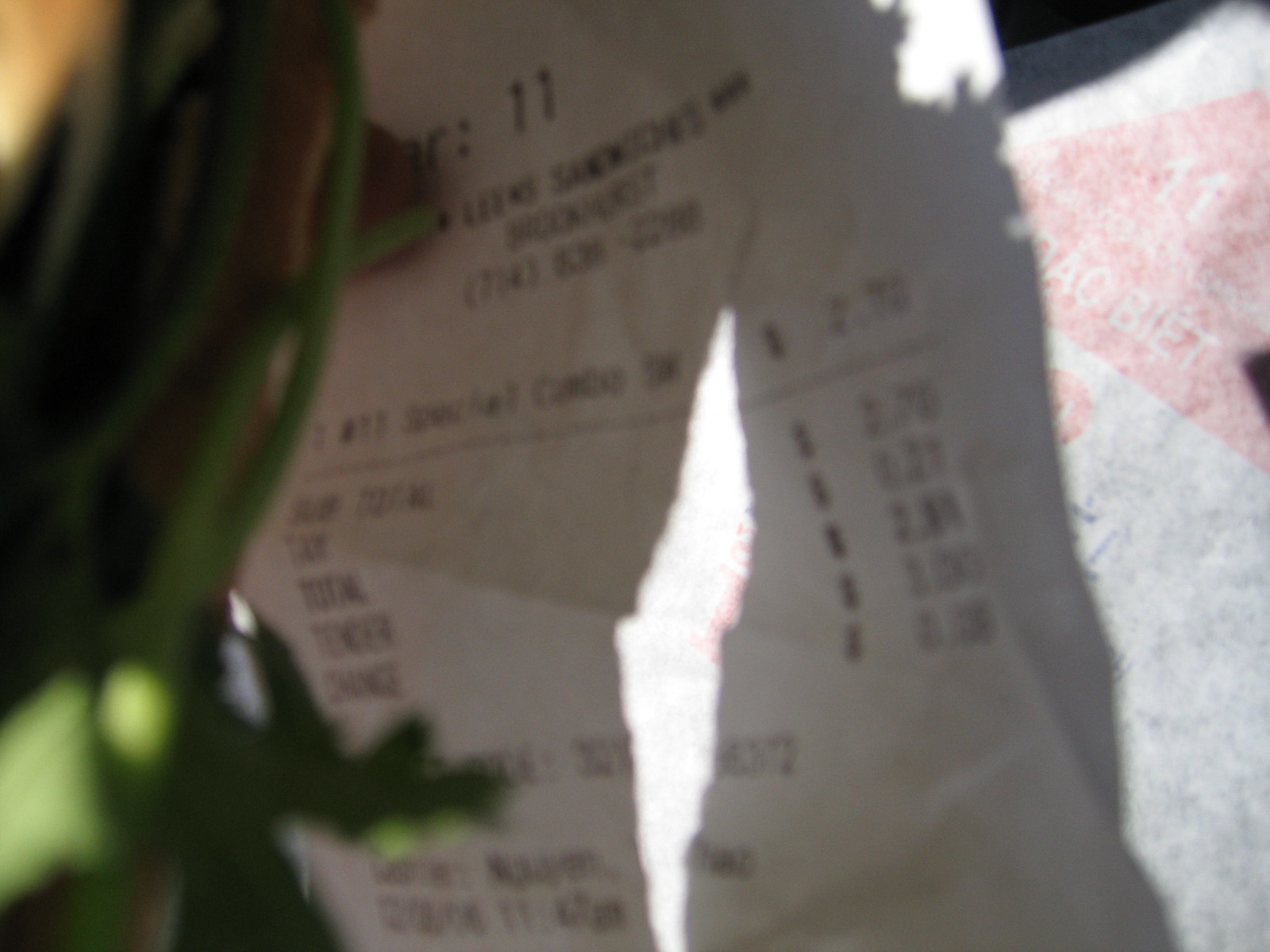The image is a close-up photograph primarily focused on a white rectangular receipt with black typing on it. The receipt appears torn down the center, making some details hard to read, but it prominently displays the number "11" at the top. Although the text is mostly blurry, it includes the company name, a phone number, and a list of purchased items along with their prices. In the left background, there's a blurry but recognizable green plant, possibly with large leaves. To the right, the background features a floor or surface with a pinkish hue and a red triangular logo. The overall scene has a dark, somewhat indistinct background that contrasts with the bright, detailed focal point of the receipt.